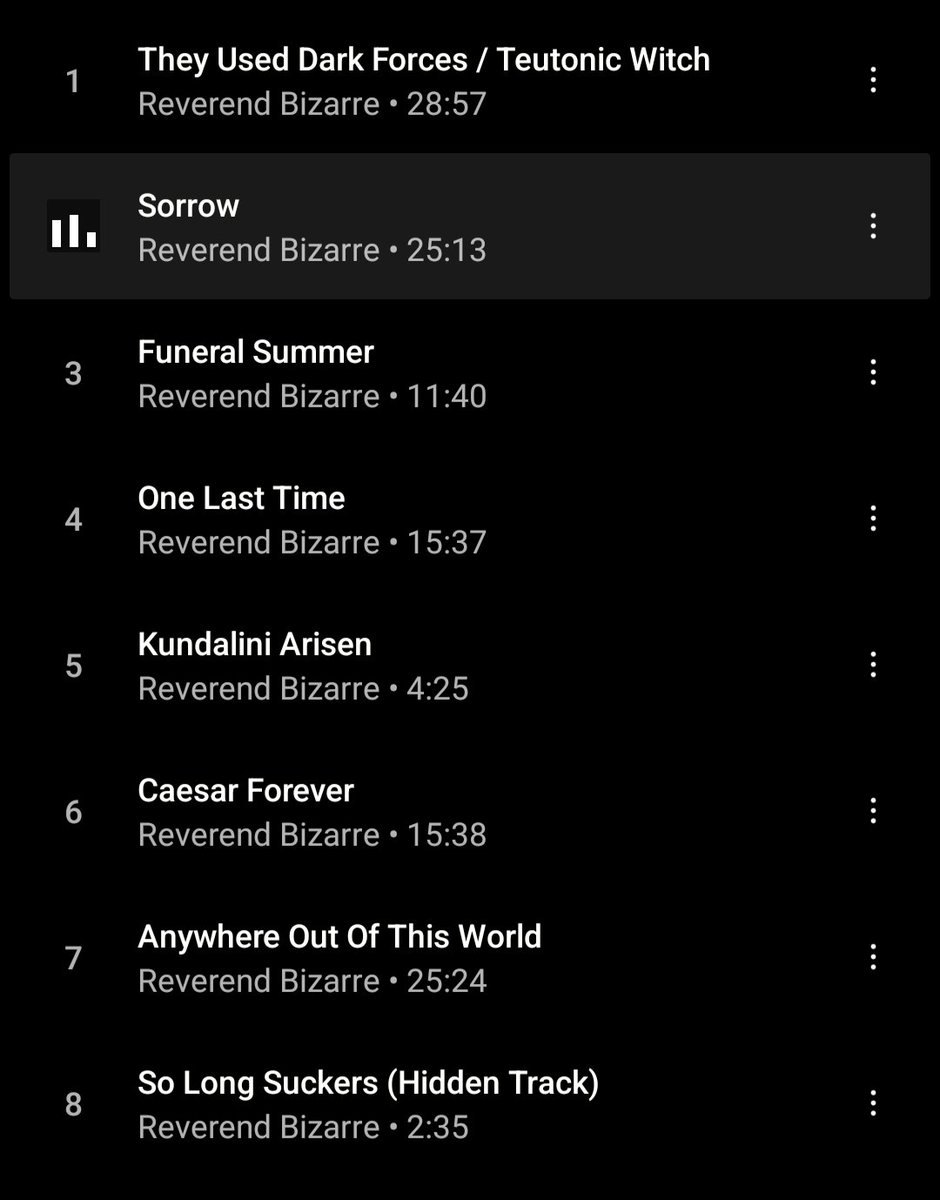The image features a solid black background, overlaid with a white text on the left side, forming a numbered list of song titles and their corresponding durations. The list is as follows:

1. **They Used Dark Forces / Teutonic Witch** - Reverend Bizarre (28:57)
2. [Indicated by a play icon, against a very deep gray background] **Sorrow** - Reverend Bizarre (25:13)
3. **Funeral Summer** - Reverend Bizarre (11:40)
4. **One Last Time** - Reverend Bizarre (15:37)
5. **Kundalini Arisen** - Reverend Bizarre (4:25)
6. **Caesar Forever** - Reverend Bizarre (15:38)
7. **Anywhere Out of This World** - Reverend Bizarre (25:24)
8. **So Long Suckers (Hidden Track)** - Reverend Bizarre (2:35)

Each title is prominently presented in a clear white font for maximum contrast against the dark background, ensuring the text is easily readable. The play icon partially obscuring number two adds a subtle visual distinction to the list, emphasizing the track's availability for immediate playback.